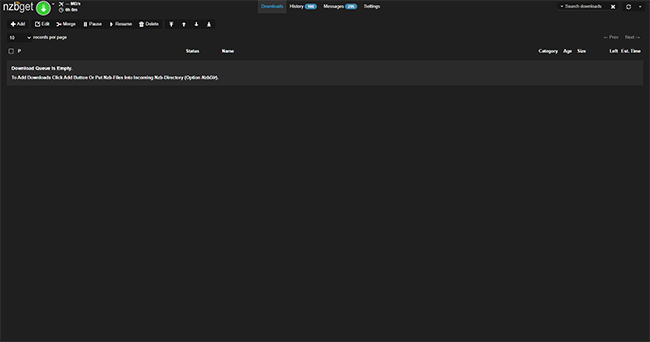The image features a predominantly black background, which appears blurry regardless of the zoom level. In the upper left corner, there's a green circle with a downward arrow next to the text "NZBGET". Centrally located at the top is a blue download button. To the right of this button, there are four clickable areas, although the labels are indistinct. Two of these areas are accompanied by blue boxes. At the top right corner, minimize and maximize buttons are visible. Below the green circle on the left, the word “Edit” is seen, accompanied by both downward and upward arrows. There are a few words beneath these arrows, but they are unclear. Further down, there's a gray rectangle with an unreadable message, followed by a blurry sentence. The remainder of the image consists of empty space.